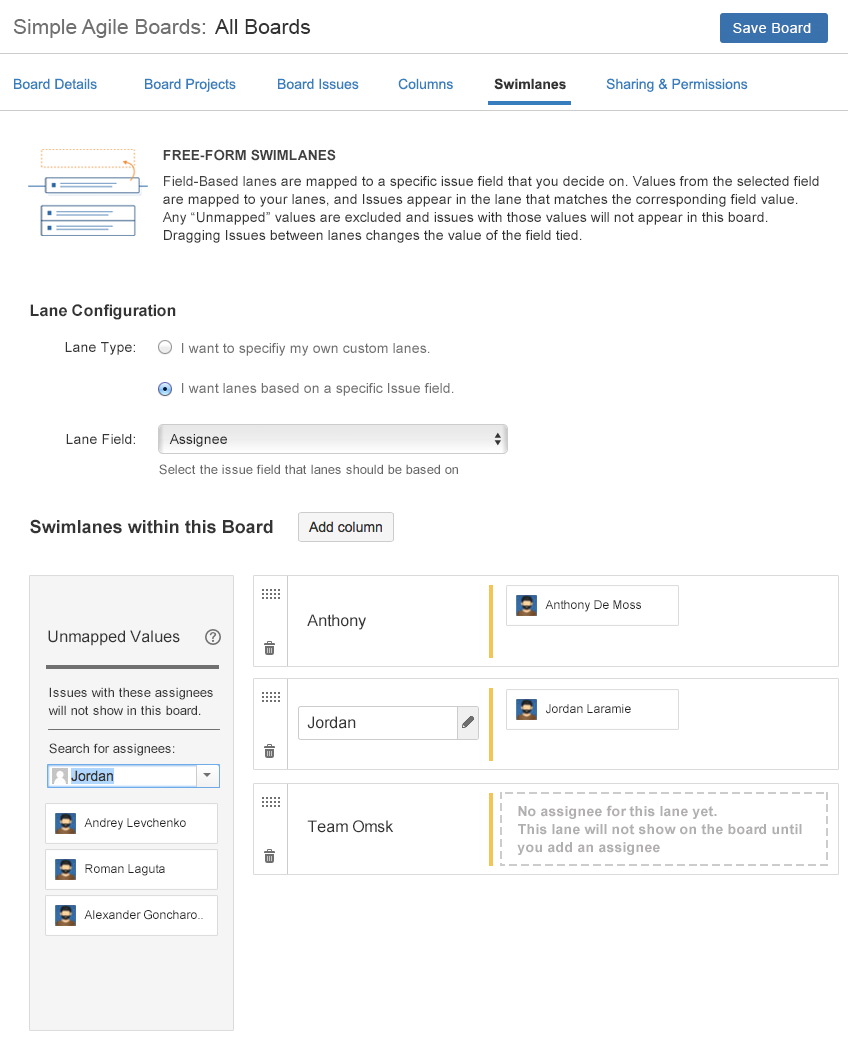The image is a screenshot of an agile project management website featuring various boards and project management tools. At the top, the header reads "Simple Agile Boards" with a sub-menu that includes options such as "All Boards," "Board Details," "Board Projects," "Board Issues," "Columns," and "Swim Lanes or Sharing and Permissions."

The main section describes "Freeform Swim Lanes," accompanied by a paragraph explaining their functionality. Key elements below this include "Lane Configuration" and "Lane Type," where the user has selected "Lanes based on a specific issue field," specifying "Assignee" as the lane field.

Underneath, the section titled "Swim Lanes within this Board" displays an "Add Column" button. The swim lanes are segmented by names at the top—Anthony, Jordan, and Team OMSK—indicating these are assignees managing different tasks or issues within the board. Additionally, the same names appear on the right side of the image, likely corresponding to specific users assigned to various tasks.